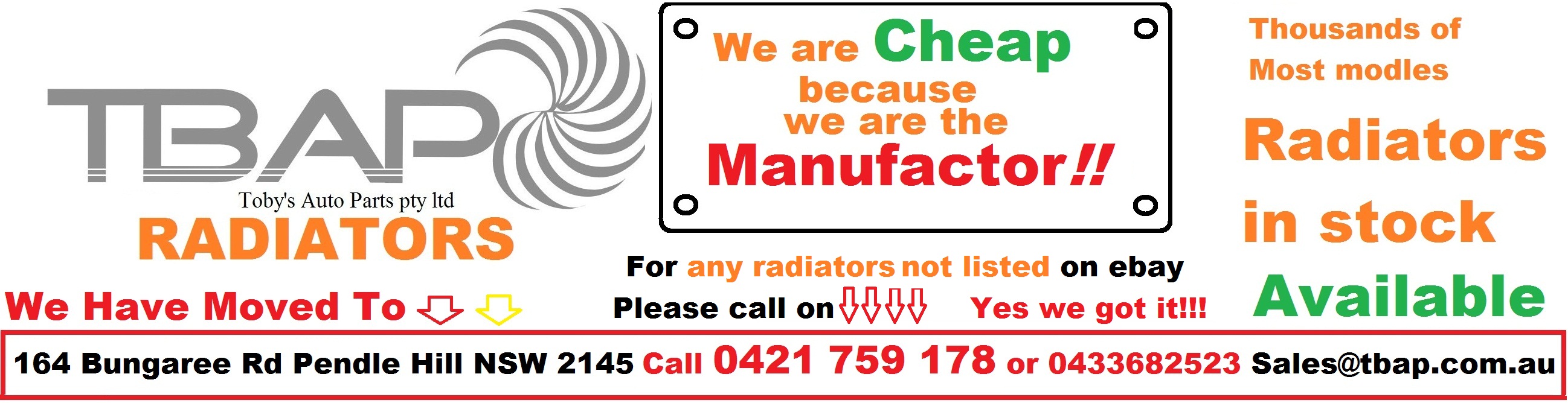The advertisement scene prominently features a central whiteboard with text and graphics. The whiteboard, secured with bolts on each corner, announces, "We are cheap because we are the manufacturer," with "cheap" in green and "manufacturer" in red, while the rest of the text is in orange. To the right, it states, "Thousands of most models," though "models" is misspelled as "M-O-D-L-E-S," followed by "radiators in stock" and "available." Below the main text, it emphasizes in orange, "For any radiators not listed on eBay," and continues in black, "please call on." Four arrows point down to the contact information.

On the left, gray text declares "TBAP, Toby's Auto Parts PTY LTD," accompanied by a circular logo of small, right-curved blades, and beneath that, "radiators" in orange. The phrase "We have moved to," with a red and yellow down arrow, leads to the new address, 164 Bungary Road, Pendle Hill, NSW 2145, framed by a thin red pinstripe. The contact information includes the phone numbers "0421-759-178" and "0433-682-523," the email "sales@tbap.com.au," and the slogan "Yes, we got it!!!" in an enthusiastic tone. The entire advertisement is set within a very thin horizontal rectangle, broad and low, providing a comprehensive overview of the company’s offerings and new location details.